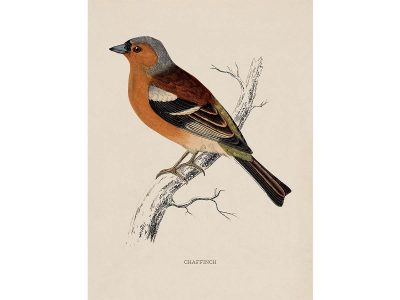This detailed illustration is of a Chaffinch bird, labeled "Chaffinch" at the bottom. The bird, depicted in a side view showing its left profile, sits on a curved branch that extends from the bottom left to the upper right of the light pink rectangular background. The Chaffinch displays a vibrant mix of colors: the bottom portion of its body is a gradient of orange to white, while the top portion, including the head, is gray. Its beak is also gray, and there is a distinct black patch between its beak and the top of its head. The wings showcase a striking pattern of black, white, and dark brown feathers with some white lines. Additionally, the bird has green feathers on its back and a black tail. Sparse leaves and buds on the branch indicate a likely winter setting, and the entire scene is monochrome except for the colorful bird.